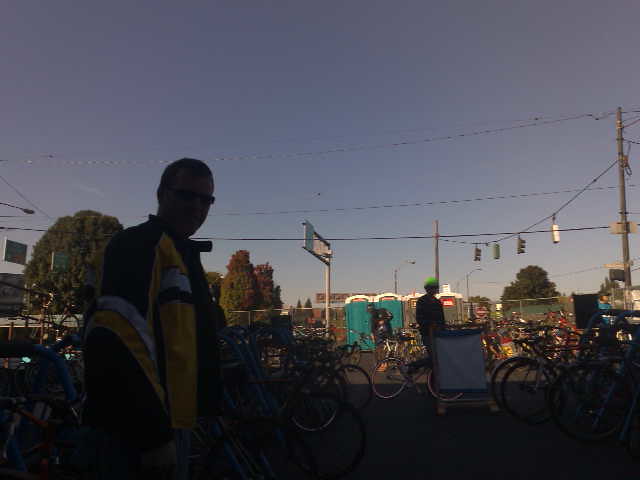The photograph captures a shaded public space during what appears to be late afternoon. Dominating the scene are multiple rows of parked bicycles suggesting a bike race or commuter lot, given the sheer volume of bikes. The sky above occupies half of the image, presenting a gradient from dark blue to lighter blue with no clouds, indicating a clear but potentially late day. In the forefront stands a man in a yellow jacket with black sleeves and white stripes, wearing dark sunglasses. He is partly turned towards the camera, with his body facing right and his head looking forward. Behind him, to the right, is a person with green hair wearing a black shirt, standing next to a bicycle. The image also includes rows of port-a-johns and a white sign that is unreadable, all set against the backdrop of a dim, shaded area with no prominent buildings or cars in sight.